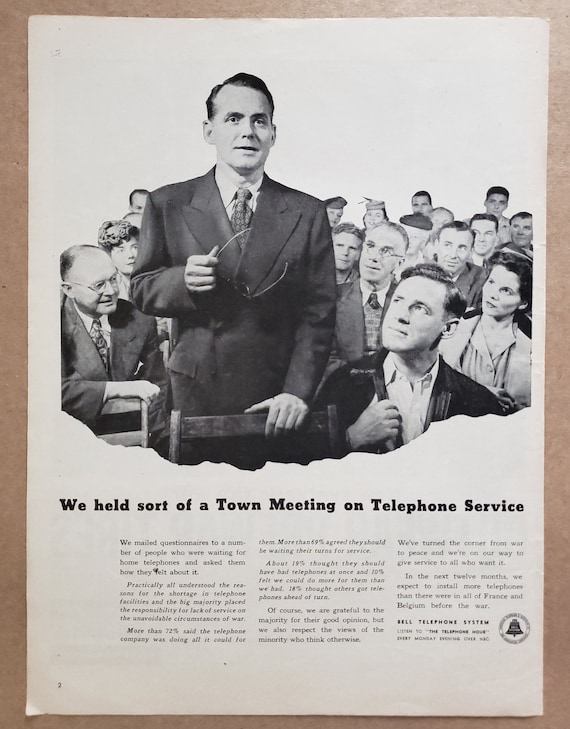The image is an old black and white advertisement for Bell Telephone, presumably from the 1940s or 1950s. The top portion features a black and white photograph capturing a town meeting setting, with a man in a suit standing up at the front, holding his glasses, with one hand resting on a chair. Surrounding him are attentive men and women, many of the men also dressed in suits. Below the photograph is a title text that reads, "We held sort of a town meeting on telephone service." The advertisement continues with three columns of text, each containing several paragraphs detailing the service. In the bottom right corner, the iconic Bell Telephone brand symbol is prominently displayed. The ad itself is printed on a white sheet of paper that has yellowed around the edges, and it is framed by a brownish hue from the visible background surface.